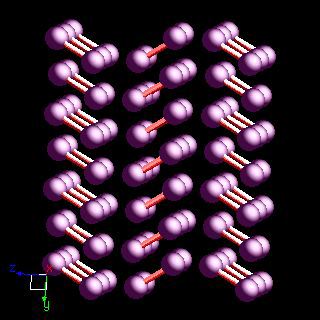The computer-generated image features a black background adorned with multiple three-dimensional structures resembling dumbbells, each composed of two purple spheres connected by a rod of varying color. These structures are arranged in three rows, each row containing alternating pairs of two and three dumbbells. In the first and third rows, the rods align diagonally down to the right, with the rods being lighter at the top and casting shadows below. The middle row features rods that are distinctly red and align diagonally upwards to the right. The image also includes a significant detail in the bottom left corner, where a blue "Z," a red "X," and a green "Y" are positioned around a white square, potentially acting as a key to interpreting the image. The meticulous arrangement and choice of colors hint at a scientific visualization, possibly representing atoms, molecules, or similar structures.